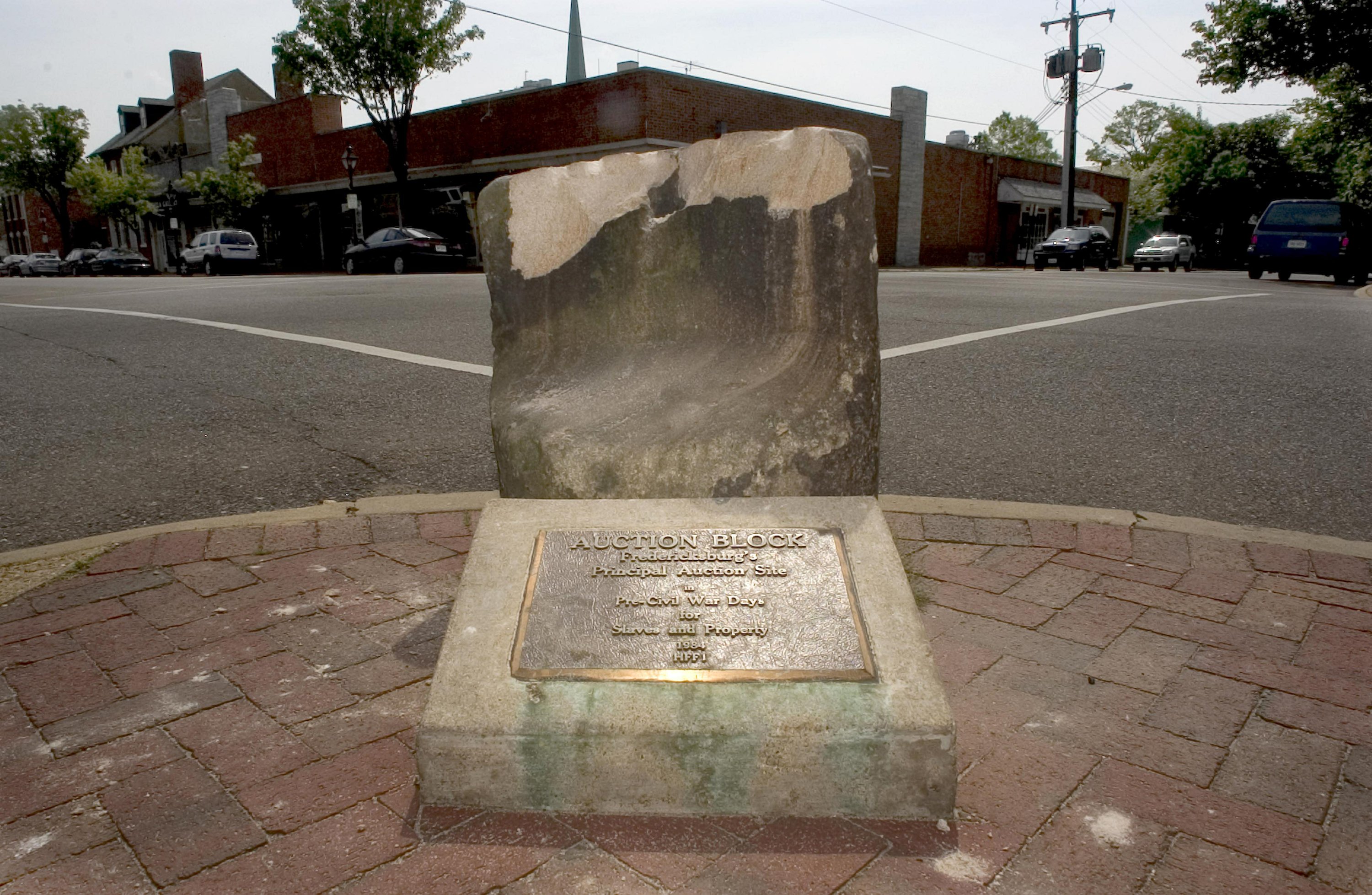This detailed image captures a defaced historical memorial or tombstone located in a downtown or suburban neighborhood area. The memorial, once an auction block, stands damaged with visible cracks and missing segments, suggesting it was struck by something heavy, possibly a car or a hammer. Inscribed on the stone is the poignant text: "Principal Auction Site in Pre-Civil War Days for Slaves and Property 1984 HFFI." Surrounded by a mix of red and grey brick pavement, this site is situated right next to the curb with a ramp for pedestrians. The background reveals a bustling street lined with brick buildings—both red and white—with cars parked in front and trees growing nearby. An awning extends over the entrance of a shop to the right, all under a bright blue sky dotted with white clouds. White road markings are visible on the asphalt, completing this snapshot of a historical yet urban setting.